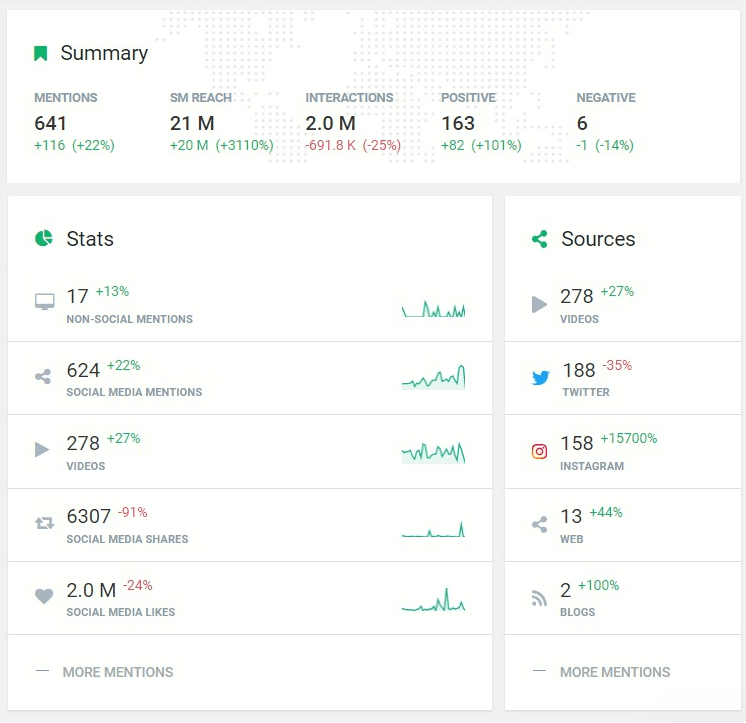The image displays various statistics and metrics in a comprehensive summary. At the top, it highlights a summary mentioning the following data:

- 641 mentions (+116)
- 22% social media reach (21 million + 20 million), with a 31% interaction rate resulting in 2.0 million interactions
- A decrease of 691.8K (-25%)
- Positive mentions: 163 (+82), representing a 101% increase
- Negative mentions: 6 (-1), representing a 14% decrease

On the left side, the statistics include:

- 17 (+13%) non-social mentions
- 624 (+22%) social media mentions
- 278 (+27%) videos
- 6307 shares (-0.1%) on social media
- 2.0 million social media likes

These metrics provide a detailed overview of online engagement, reach, and sentiment.